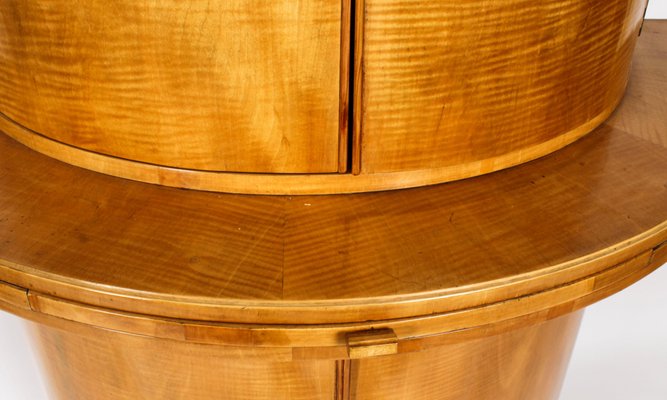The image depicts a close-up of a handmade wooden piece of furniture, likely a desk or a specialized counter for a self-service area, such as one used to prepare checks in a bank lobby. The furniture features a circular frame with a smoothly finished, light maple or honey-brown colored wood, accentuated with a highly polished and sealed surface, possibly coated with clear varnish. The top section includes a narrow, round shelf inset with a plexiglass layer, and the curvature reveals seams indicating the sectional assembly of the piece. Centrally on the side, there is a handle which might be used to pull out or adjust a section to widen the surface area. Despite the zoomed-in perspective cutting off parts of the furniture, the visible sections highlight the detailed craftsmanship and the natural wood grain, set against a white background.